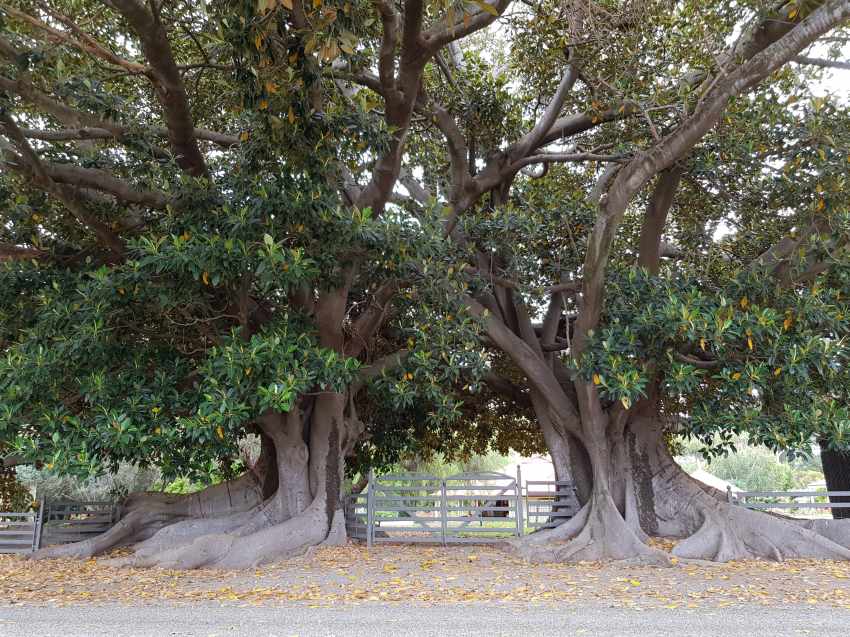The image captures two immensely imposing, picturesque trees with a distinctive weeping willow-like appearance, their pronounced and well-established trunks detailed with visible, sprawling roots that almost seem to dive into the ground. Positioned a few feet apart, the trees create an arch-like structure with their thick, intertwined branches, suggesting they have been part of the landscape for a long time. The ground beneath them is a mix of gravel and concrete, scattered with early-fall leaves that are turning golden and orange while most of the foliage remains green. Between the trees, there is a path leading to a closed gate, part of a wooden fence that stretches out behind them. In the distant background stands a white, ranch-style house with a hipped roof and an open garage door, framed by a cloudy white sky visible through the branches. A thin sliver of a gravel road runs across the bottom of the picture, emphasizing the courtyard-like feel of the setting, possibly indicative of a place where horses could be kept and run.